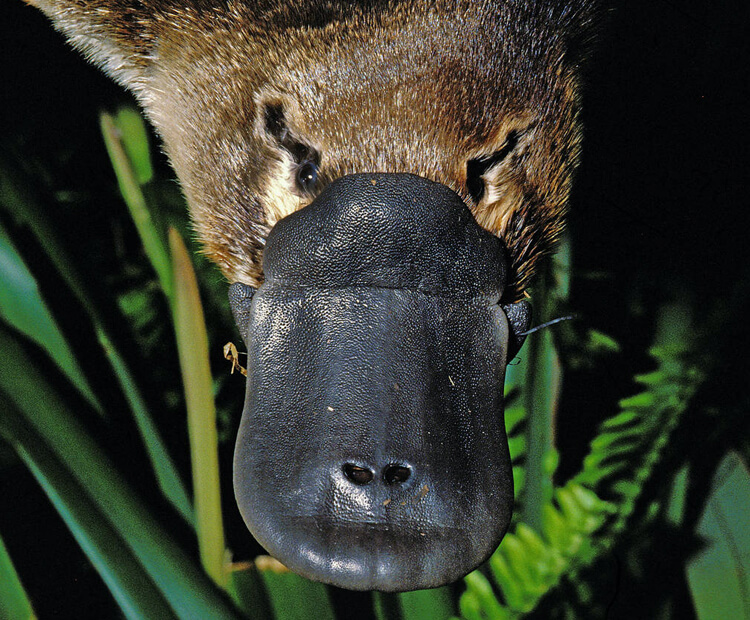In this captivating image, a duck is prominently featured, showcasing its rich, brown plumage that gives it a warm, earthy appearance. The duck's two black eyes are strikingly set against its feathered face, exuding alertness and curiosity. Its beak, a distinctive elongated oval shape and entirely black, draws immediate attention. Near the tip of the beak, there are two heart-shaped nostrils, adding an intricate touch to its facial structure. The background is filled with verdant green shrubs, plants, and leaves, creating a lush, natural setting that is slightly dimmed, focusing the viewer's attention on the foreground subject. The duck appears to be gazing attentively, adding a dynamic quality to the scene.